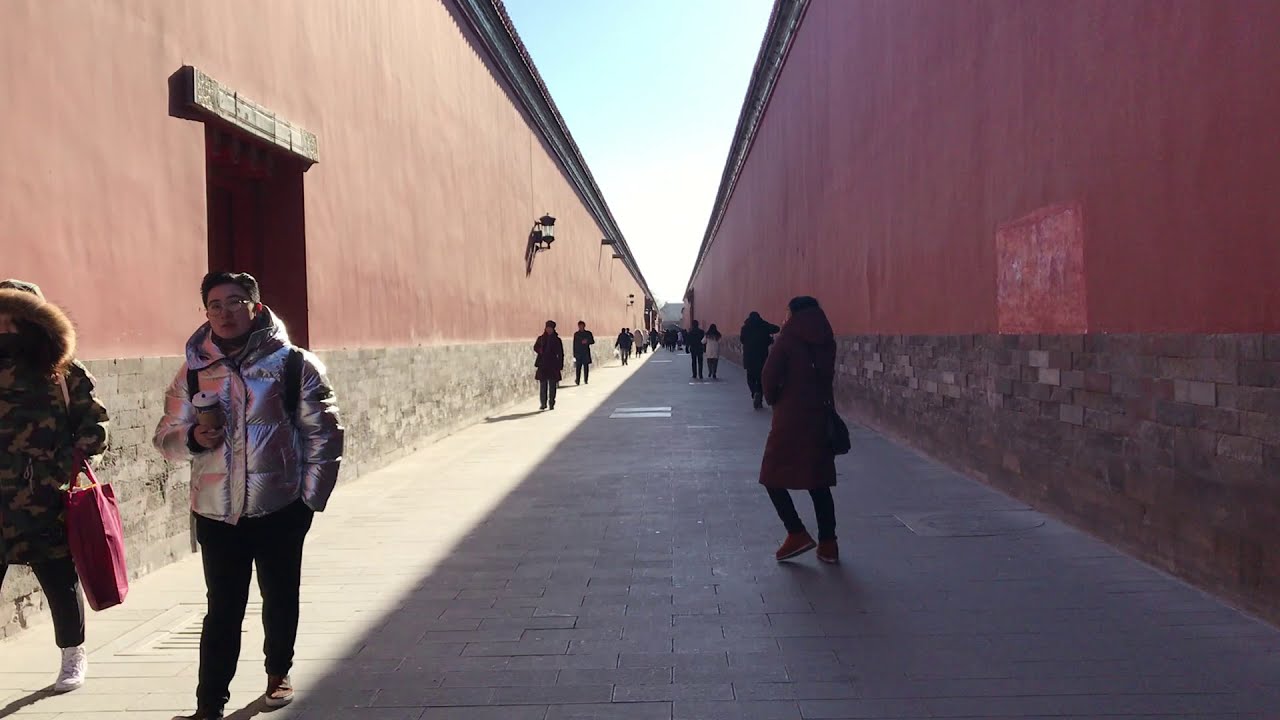The horizontally aligned landscape photograph captures a bustling, wide alleyway with a stonework path set between two red buildings that have beige brick foundations up to chest height and tall red walls above. A blue sky with scattered white clouds peeks through the top middle of the frame. In the foreground on the left, a man with short black hair, wearing eyeglasses, a silver puffy jacket, and black pants, holds a coffee cup in his right hand. Next to him further left, a woman dons a camouflage hooded jacket with brown-fur trim, black pants, and carries a red bag over her left arm. Both of these figures, along with a crowd of others in the background moving in both directions, illustrate the lively comings and goings on this pathway. Decorative elements include lights mounted on the left building's wall and a doorway just behind the coffee-holding man, possibly hinting at the alleyway being part of a building. Additional details include a repainted patch on the right building's wall and a sign with foreign text above one of the doorways on the left. The photograph exemplifies realism with its detailed depiction of the urban outdoor scene.